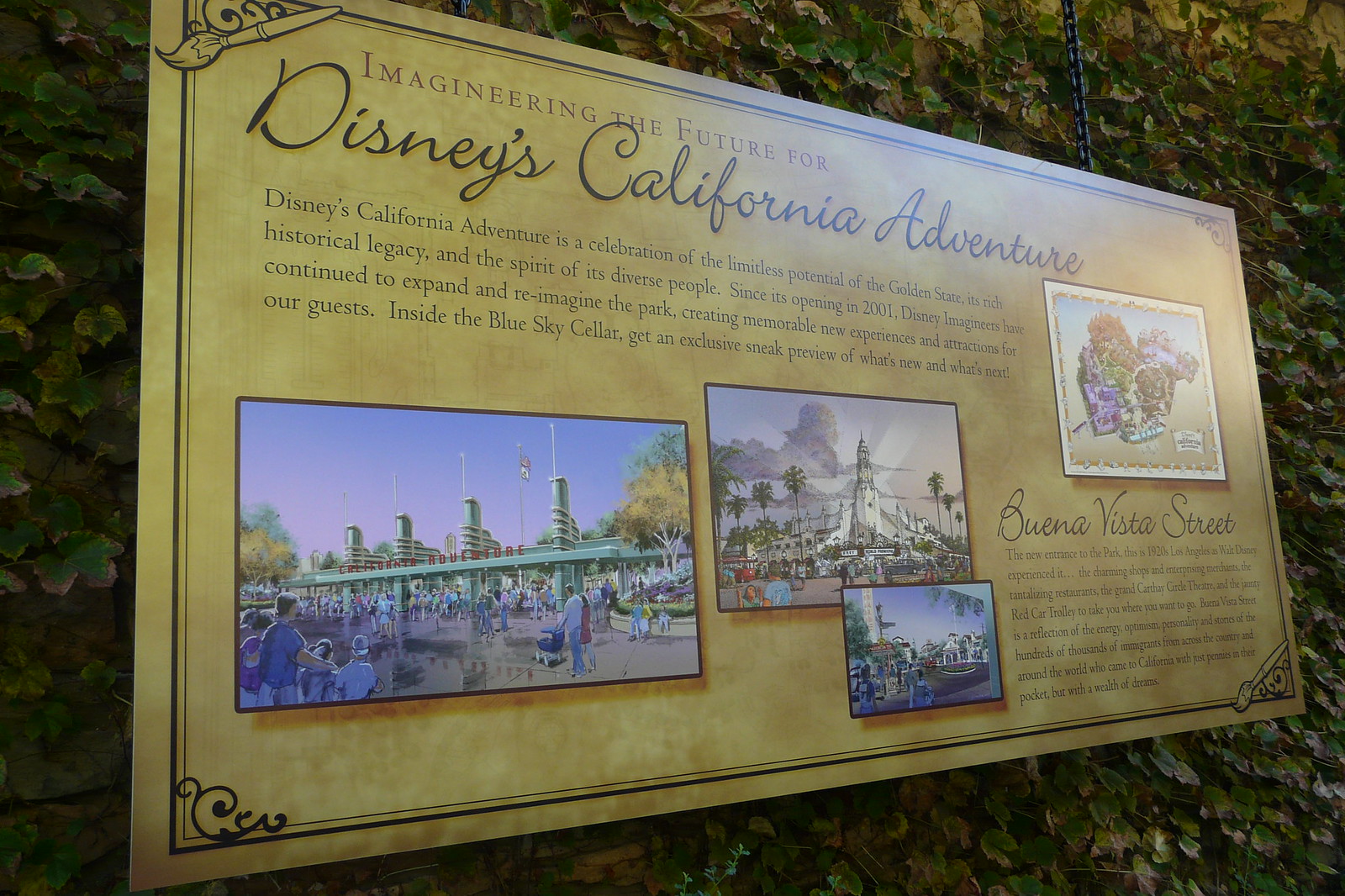This detailed, full-color photograph captures a sign being hung by black chains, positioned against a backdrop of a stone wall. The sign itself is predominantly brown with gold accents and is adorned with four artistic renderings that provide a glimpse into the conceptual design for Disney's California Adventure.

The primary text on the sign reads, "Imagineering the Future for Disney's California Adventure," with "Disney's California Adventure" elegantly scripted in cursive. Additional cursive text highlights "Buena Vista Street." The sign proclaims that Disney's California Adventure is a celebration of the limitless potential of the Golden State, acknowledging its rich historical legacy and the spirit of its diverse people since the park's opening in 2001.

A detailed description continues on the sign, stating how Disney Imagineers have continually expanded and reimagined the park, creating new memorable experiences and attractions. It invites guests to explore the Blue Sky Cellar for an exclusive preview of future developments. At the bottom right, more text describes Buena Vista Street as the new entrance, designed to evoke 1920s Los Angeles as Walt Disney himself experienced it, with charming shops, enticing restaurants, the Grand Carthy Circle Theater, and the Red Car Trolley.

Buena Vista Street symbolizes the energy, optimism, and stories of numerous immigrants who arrived in California with scant resources but grand dreams. The sign, portrayed through artistic renderings, hints at a nostalgic yet innovative reimagining of the park's entrance, reflecting the imaginative future Disney continues to build.